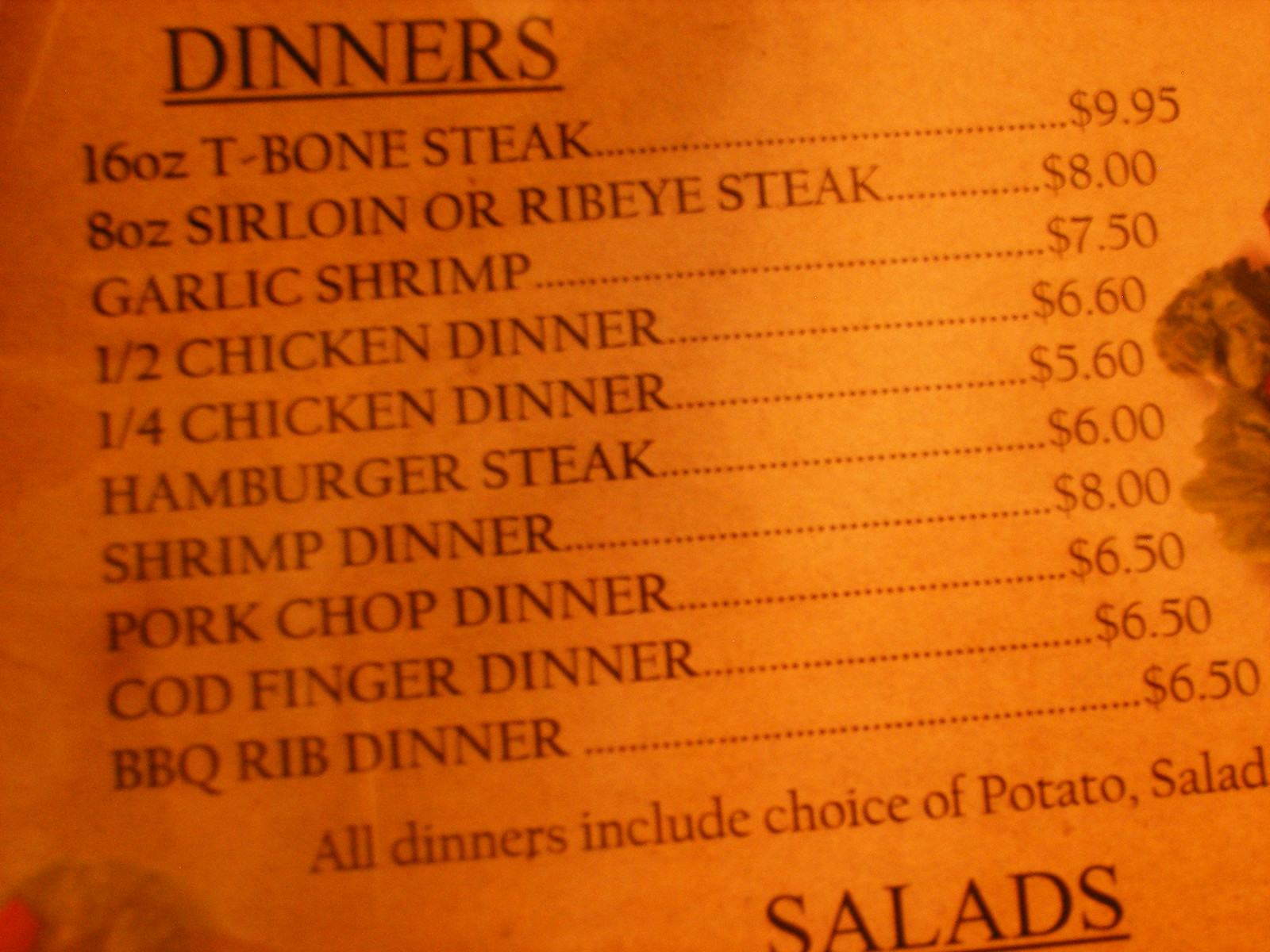This image depicts a dimly-lit, poorly-captured photograph of a menu printed on dark-colored paper with black ink. At the top of the menu is a header labeled "Dinners." Listed below are various meal options:

- 16oz T-bone steak - $9.95
- 8oz sirloin or ribeye steak - $8.00
- Garlic shrimp - $7.50
- Half chicken dinner - $6.60
- Quarter chicken dinner - $5.60
- Hamburger steak - $6.00
- Shrimp dinner - $8.00
- Pork chop dinner - $6.50
- Cod finger dinner - $6.50
- Barbecue rib dinner - $6.50

At the bottom of this list, there is a partially cut-off text that reads "All Dinners Include Choice of Potatoes, Salad, and..." The details beyond this point are obscured. Below this incomplete message, another header titled "Salads" marks the end of the visible portion of the menu.

On the far right side of the menu, there appears to be an image, possibly of food like broccoli, though it could also be a stain. The bottom left corner of the image shows what looks like a finger, suggesting someone is holding the menu.